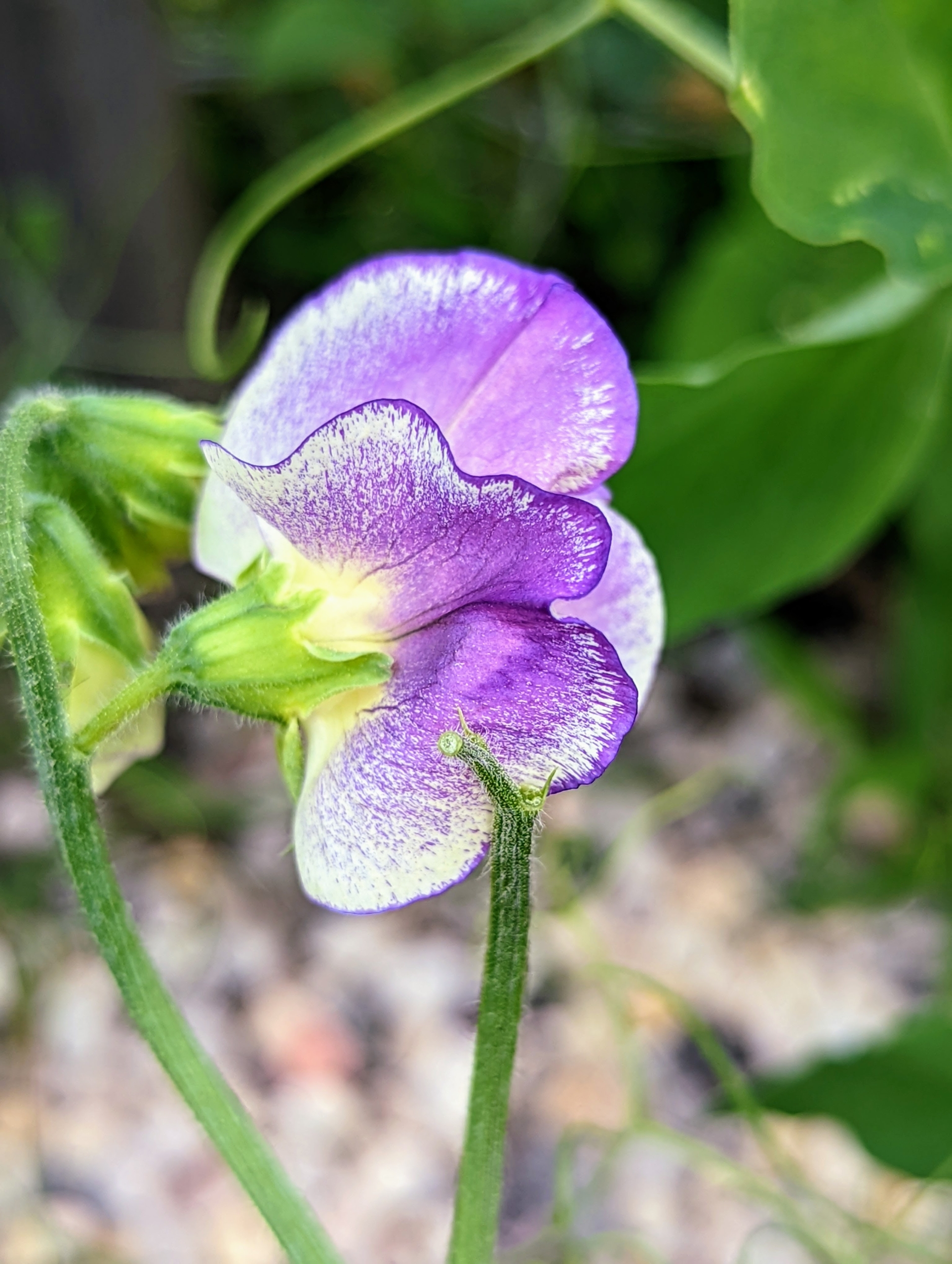The image presents an extreme close-up of a beautiful, delicate purple and white flower with intricately curved edges and veins of deep purple that accentuate its petals. The flower begins with a speckled white center, transitioning to a vivid purple with dark edges. It stands on a light green, somewhat fuzzy stem, accompanied by another stem that branches off to the left. The background of the photograph is a blur of greenery and additional leafy plants, emphasizing the flower’s detail. At the bottom of the image, a speckled gray-white area hints at a stony surface, grounding this exquisite bloom. Behind the main flower, there is a slightly larger purple flower, adding depth and context to this intricate natural scene.